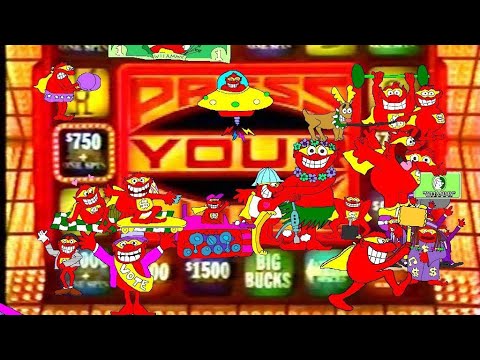The image is a highly detailed and vibrant still from what appears to be a cartoony arcade or gambling game. The central square reads "Press Your Luck" or "Press U," surrounded by various dollar amounts like $750, $1,500, and captions such as "big bucks." Dominating the scene are dozens of small, red, humanoid characters, each uniquely costumed and animated. One character is featured in a yellow flying saucer, another is lifting a green dumbbell, and a third is smiling broadly and seems to be yelling. Some wear capes, boxing gloves, or hula skirts. Notably, one character wears a yellow sash with "VOTE" written in white letters. The scene also incorporates a vivid array of colors, including red, yellow, green, blue, purple, and pink, with some black and white accents. The overall composition suggests a chaotic yet playful environment, reminiscent of a whimsical fever dream.